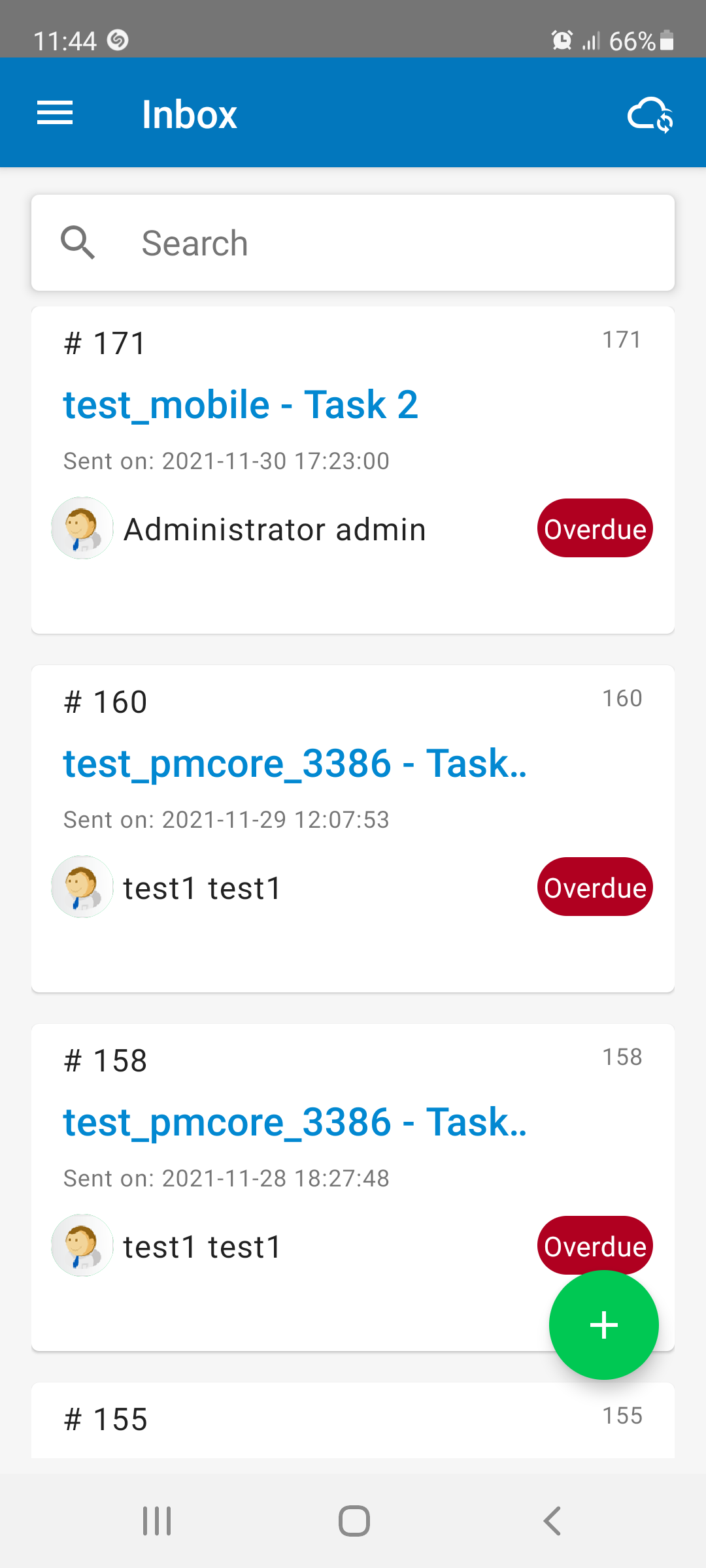The image depicts a screenshot of someone's inbox on their phone. At the top of the screen is a gray rectangle, followed by a blue rectangle, and at the bottom is a very faint gray rectangle containing long and skinny white rectangles. Inside this bottom area is a search bar featuring a magnifying glass icon and the word "Search."

The inbox lists several tasks:
1. The first task, listed as "test_underscore_mobile-task 2," is labeled number 171 and assigned by "administrator admin." It is marked as "overdue" within a red, circular notification on the right, and there is a generic avatar icon on the left.
2. The second task, labeled "number 160," is titled "test PM core_3386-task..." and features "test 1 test 1" beneath it. This task also has a red overdue notification.
3. The third task, labeled "test PM core_3386" and numbered 158, is similarly marked as overdue. Additionally, there is a green circular icon with a plus sign on it.

The list appears organized by task number, with overdue notifications clearly highlighted in red circles on the right side of each entry.